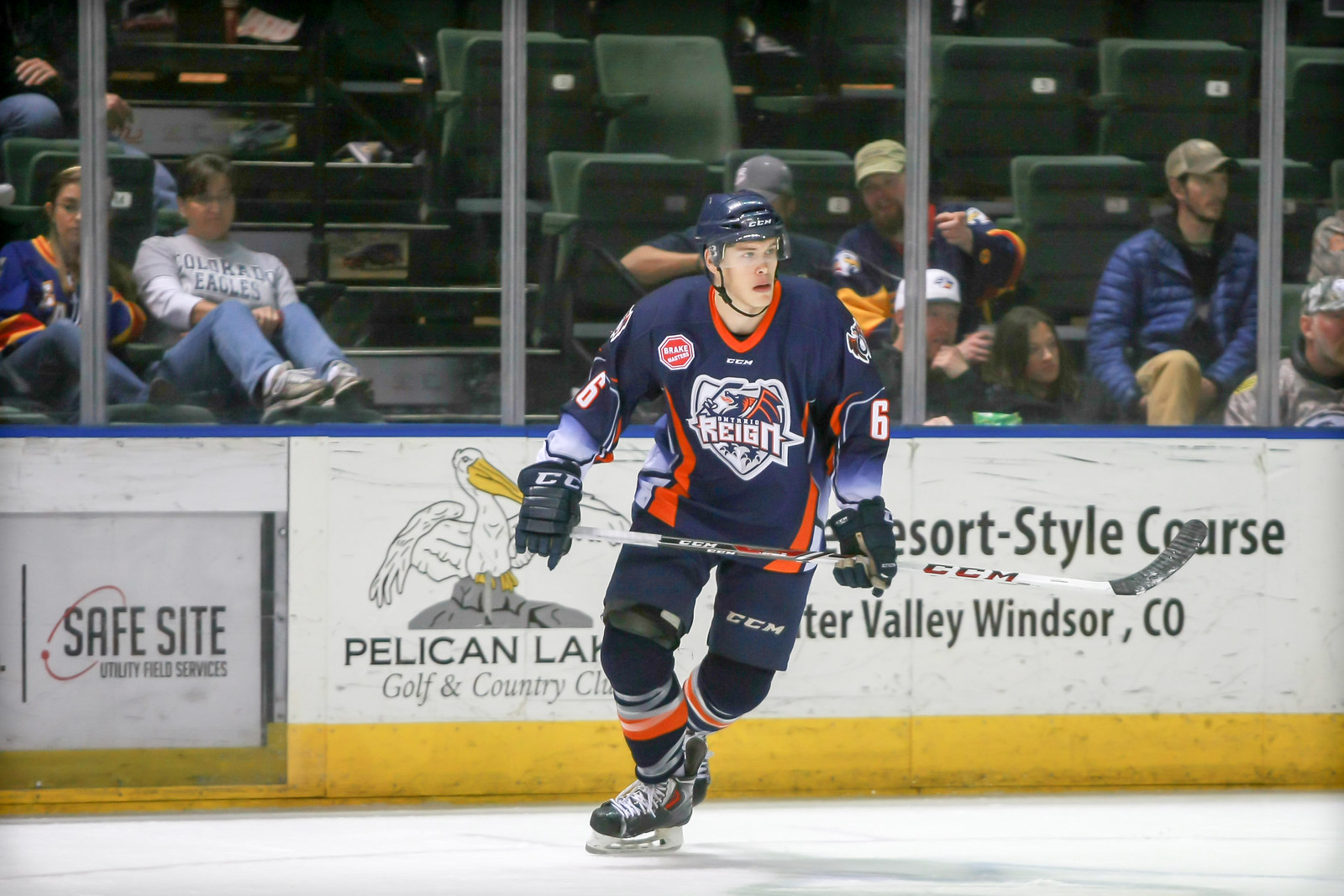This is a detailed, color photograph capturing a moment from a hockey game, presented in landscape orientation. The central subject of the image is a single hockey player mid-action on the ice rink. The player is framed in the middle of the image, skating toward the left while looking away towards the camera. He is wearing a blue jersey with distinctive orange stripes and a logo in the center that reads "Rain" (spelled R-E-I-G-N). Complementing his jersey are navy shorts and hockey skates. The player is in motion, with his right foot forward and left foot back, pushing off the ice while holding his hockey stick across his midsection.

In the background, the photo includes a partition split into a top half of plexiglass and a bottom half covered by a banner with sponsor logos. On the left side of the banner, there’s an advertisement for "Safe Light" with a corresponding logo. Just right of this, another ad for "Pelican Lake Golf and Country Club" features a cartoon pelican; additional text denotes it as a resort-style course located in Windsor, Colorado. Beyond the partition, viewers are seated in the stands, attentively watching the game. The overall style of the image leans toward photographic representationalism realism, capturing both the dynamic action of the hockey player and the vivid details of the surrounding environment.